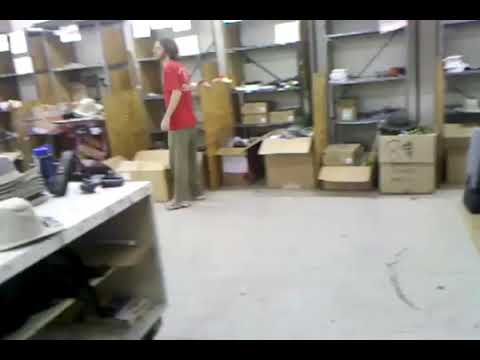The photograph captures a scene inside a warehouse with a thin black border at the top and bottom. The focal point is a young man with short black hair, standing and facing left. He is wearing a red T-shirt and light gray pants. The warehouse is characterized by a light gray or beige linoleum floor, devoid of any tile grid patterns and slightly shiny. The background reveals a long row of steel shelves along the back wall, cluttered with various items, cardboard boxes, and papers. In front of these shelves are large cardboard boxes, seemingly full though their contents are not visible. To the left of the man, there is a white marble desk with two shelves, holding miscellaneous items such as a ticket machine, a pricing gun, and a white hat on top. The walls of the warehouse are gray, and there are some light sources at the top, possibly square, bare windows. The overall setting appears somewhat disorganized, typical of a busy warehouse environment.